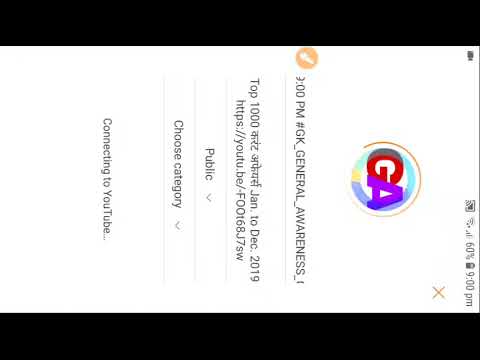The sideways image, resembling a screenshot, features a white central section flanked by black borders on the top and bottom. At the top right in the correct orientation, it displays "9 p.m." along with small icons indicating internet connection and battery life. In the center, there is a multicolored circular logo with the letters "GA," where "G" is red and "A" is purple, surrounded by a blue circle outlined in red. Below the logo, the main text reads "9 p.m. GK general awareness," followed by "top 1000" and "January to December 2019." An HTTPS YouTube link (HTTPS://YouTube/FD0068.17SW) is listed beneath. Further down, there are options for "public" and "choose category," each with adjacent downward arrows, and the text concludes with "connecting to YouTube." The image, which needs a 90-degree counterclockwise rotation to be read correctly, includes an "X" icon and a movie camera symbol to the left, indicating potential navigational or functional options.